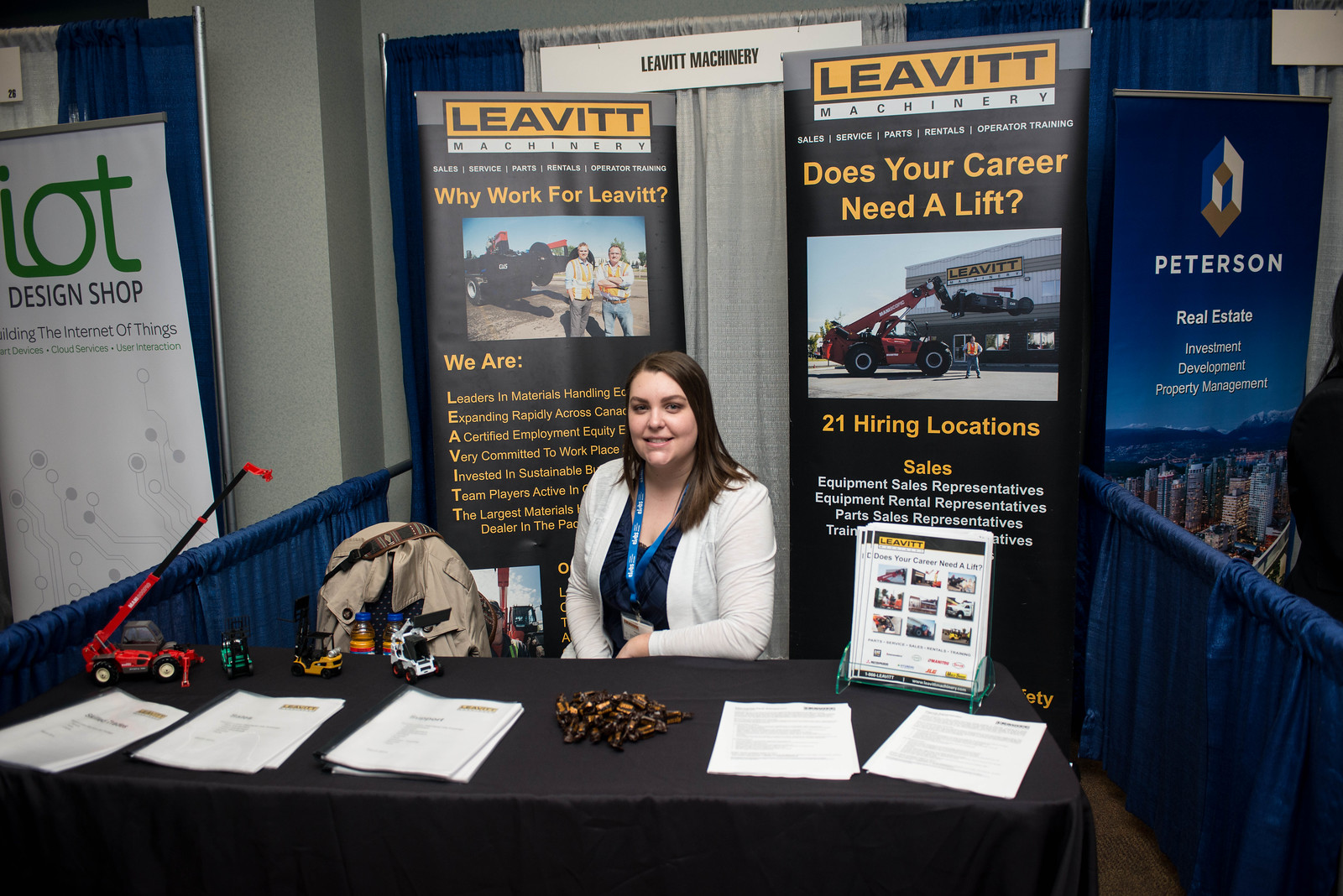The photograph captures a woman seated at a booth during a business conference. She is wearing a white jacket over a blue dress and a blue lanyard with a laminated identification tag around her neck. Her hair cascades past her shoulders. The table in front of her, draped with a black tablecloth, features various objects including a central pile of candies, multiple stacks of papers, predominantly white, and an assortment of colorful toy trucks in red, green, yellow, and white. To her left, additional items and notices are displayed on the table. 

Behind her, two large vertical signs prominently showcase the company she represents, Leavitt Machinery. The sign on the right boldly states, "Leavitt Machinery. Does your career need a lift?" accompanied by an image of a large machine and further text detailing opportunities for 21 hiring locations, focusing on sales equipment representatives, equipment rental representatives, and parts sales representatives. To the left, another sign reads, "Why work for Leavitt." The background is divided by a blue sheet, indicating neighboring stalls possibly belonging to other companies, including mentions of Peterson Real Estate and a design shop.